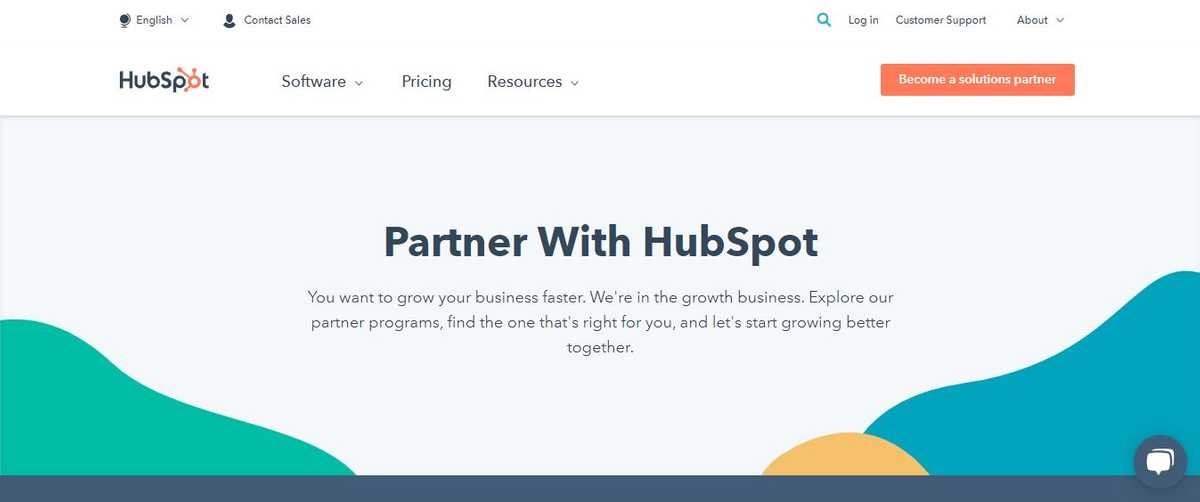Web page screenshot description: 

The web page exhibits a minimalist design with a predominantly white background. At the top center, the word "English" is displayed in black text, followed by a "Contact Sales" link. On the top-right corner, a teal magnifying glass icon denotes the search function, accompanied by several other buttons: "Login," "Customer Support," and "About," the latter featuring a drop-down arrow.

On the top-left, the HubSpot logo is prominently shown, with the 'O' uniquely colored in orange. Adjacent to this, a gray drop-down button labeled "Software" is visible, followed by similarly styled buttons for "Pricing" and "Resources." Further to the right, a vibrant orange button with white text invites users to "Become a Solution Partner."

A prominent feature is a large off-white rectangle with blue undertones, displaying the headline "Partner with HubSpot" in bold blue text. Beneath this, a dark gray subheader reads, "Do you want to grow your business faster? We're in the growth business. Explore our partner programs, find the one that's right for you, and let's start growing together."

On the left within this rectangle, a teal-colored mountain image is shown, while the right side features a dark blue mountain. Between these mountains, an orange half-circle resembling a rising sun is artistically rendered. 

The page footer is highlighted by a dark blue banner, shaped as a rectangle and complemented by a dark blue circle containing two white chat bubble icons, symbolizing communication or live chat support.